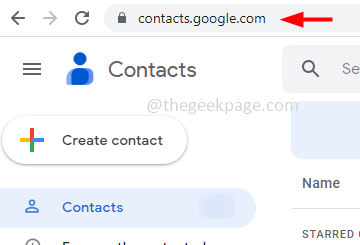The image depicts a low-resolution and somewhat pixelated screenshot of a web page, specifically a Google Contacts interface. Despite the blurriness, several key elements can be identified. In the top left corner, there are three buttons: a back button, a forward button, and a refresh button. Adjacent to these buttons is a search bar containing a lock icon and the URL "contacts.google.com." To the right of the URL is a distinctive red arrow pointing to the left.

Below this section, on the left side, a more icon and a profile icon are visible, with the text "Contacts" written next to them. Slightly to the right, a search bar is partially visible, displaying a search icon on one side. Further down, a prominent button labeled "Create Contact" is situated on the left, featuring a multicolored plus sign that includes shades of red, blue, and green.